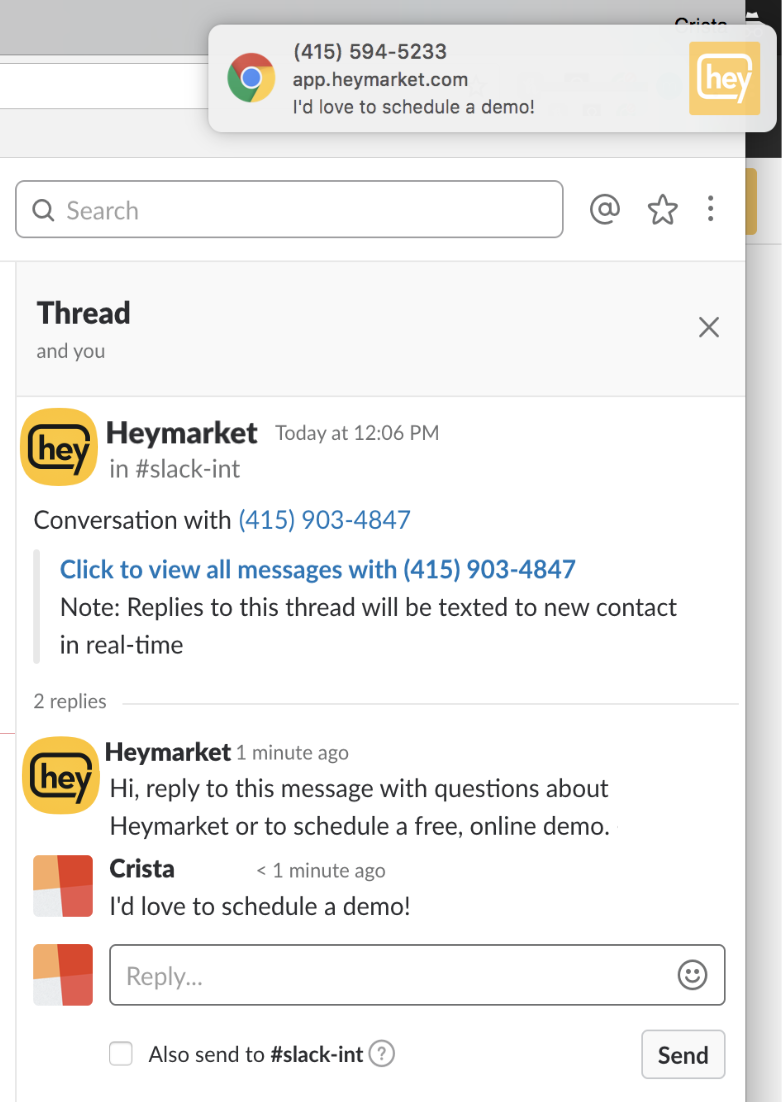In this detailed screenshot from a tablet device, we see an interface related to the Haymarket app. At the very top, a pop-up is visible displaying a phone number with area code 415-594-5233, along with the URL app.haymarket.com. The message within the pop-up reads, "I'd love to schedule a demo," accompanied by the Haymarket emblem positioned on the upper right of the pop-up.

Beneath the pop-up, there's a search bar with the label "thread and you." To the right of this label is an 'X' button allowing the user to close this section. Below the search bar, the interface shows two messages pertaining to Haymarket. The first message is timestamped "today at 12:06 PM" and is located in the #slack-int channel, detailing a conversation with the phone number 415-903-4847. This message includes a link in blue text stating, "click to view all messages with 415-903-4847," and notes that replies to this thread will be texted to new contacts in real-time.

The first reply in the thread is from Haymarket, posted one minute ago. The reply reads, "Hi, reply to this message with questions about Haymarket or to schedule a free online demo." Following this is a message from a user named Krista, also posted one minute ago. Krista's icon, featuring colors of red, dark pink, orange, and grey, is visible to the left of her message. Krista's message reads, "I'd love to schedule a demo!" Below her message, there is a reply field where Krista can type additional responses. To the far right of this field, there is an emoticon choice option. Beneath the reply field, an unchecked checkbox labeled "also send to #slack-int?" is available, accompanied by a send button.